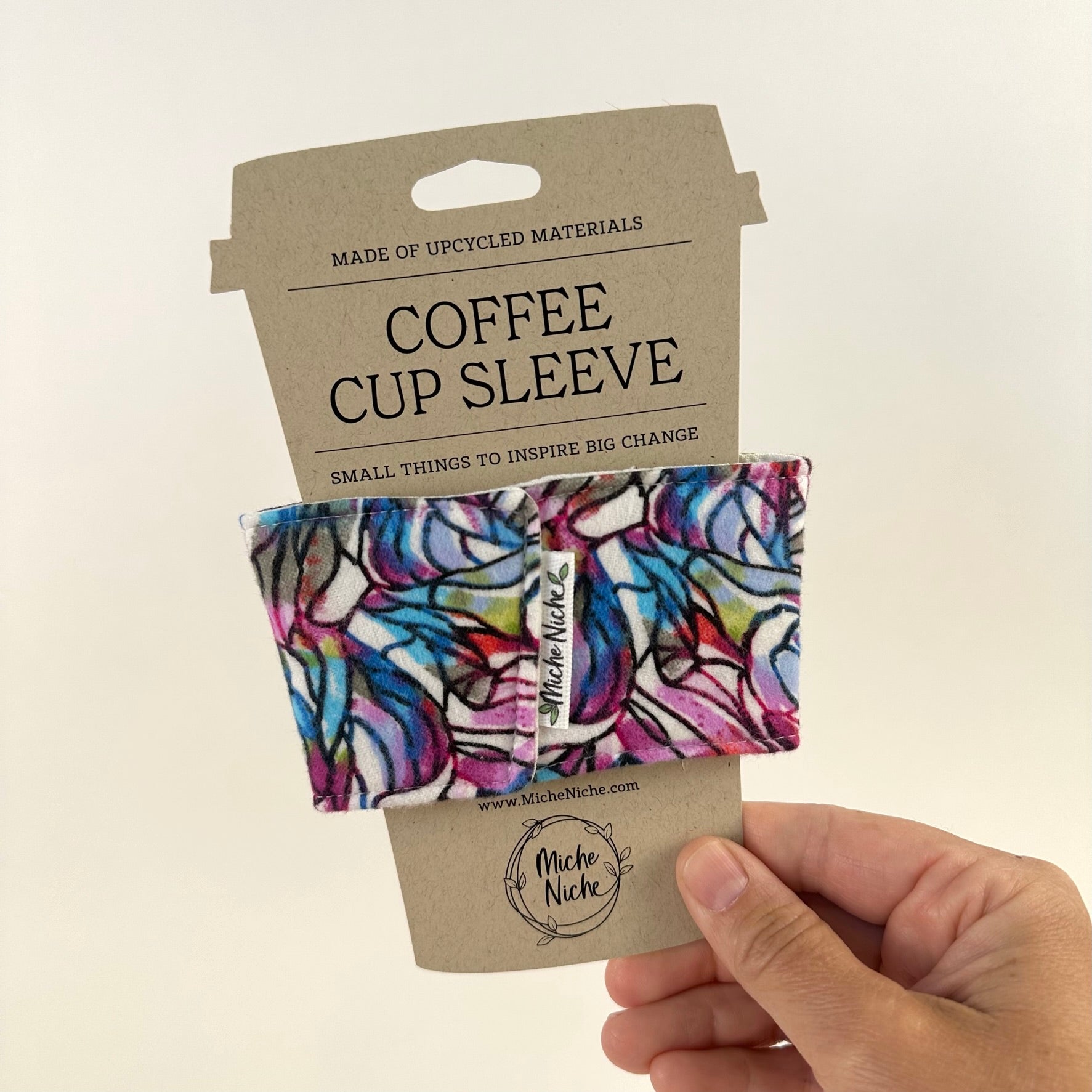In this detailed image, a hand is seen at the bottom right corner, holding up a cut-out, brown, paper coffee cup sleeve against a light beige or cream background. The sleeve is presented on a placard with a small hanger indicative of a retail display. The sleeve itself is made from upcycled materials and serves the purpose of insulating a coffee cup. The text reads in a bold font, "Made of up-recycled materials. Coffee cup sleeve." Just below a thin horizontal line, it states, "Small things to inspire big change." Towards the bottom of this placard, the website "www.micheniche.com" is repeated multiple times for emphasis. The brand name "Michnich" appears within a circular logo that also features small leaf designs around its edges. The center section of the sleeve is adorned with a multicolored fabric strip containing shades of blue, purple, black, red, white, green, and gray. The fabric boasts irregular, rectangular patterns, creating a visually appealing design.